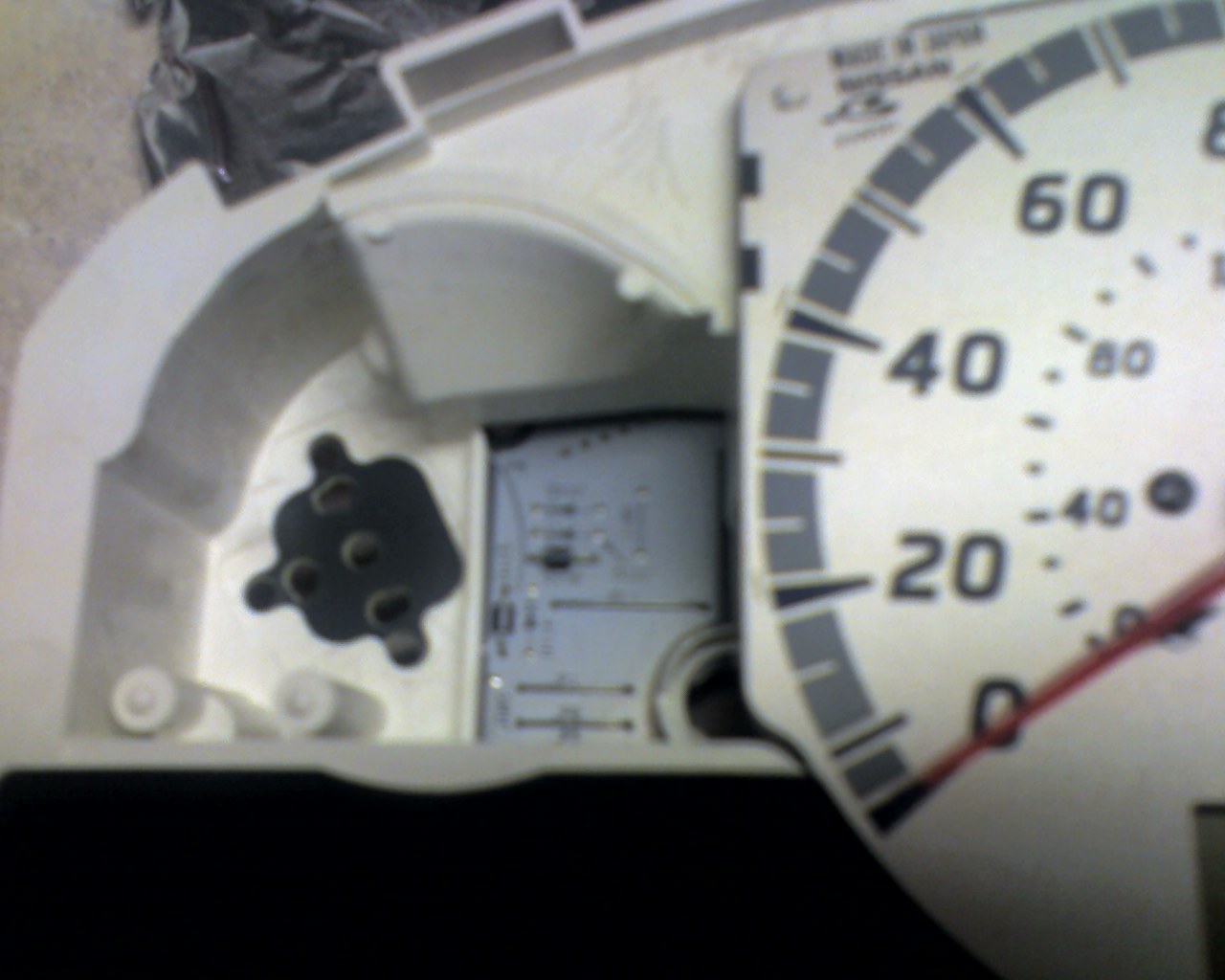This is a close-up, albeit out-of-focus and fuzzy, image of a presumably plastic dial, which appears to be part of an electrical meter. The round dial dominates the right half of the image, featuring numerals 0, 20, 40, 60, and partially 80, encircled by a black band around its circumference. The dial is characterized by its squared-off top and left sides, with the bottom remaining rounded. An inner dial, partly obscured by a red needle pointing towards what seems to be 0, displays additional markings at 40 and 80, alongside some gradient markers. On the left side of the photo, a light gray, curved, and approximately two-inch deep plastic container is visible. At the bottom of this container, there is a small black rectangle with four holes and tabs extending in three different directions.